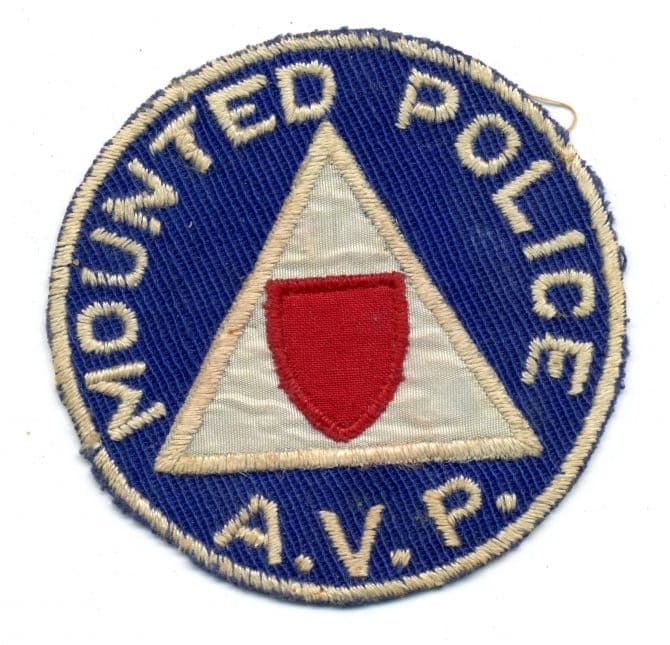The image depicts a close-up of a vintage, circular cloth badge against a pure white background. The badge, which appears worn and used, is designed for sewing onto clothing or uniforms. It has a blue fabric base with a cross-stitched pattern, and its border is intricately embroidered with a light beige thread. This beige border encircles the patch completely.

Central to the badge is an embroidered equilateral triangle made from cream-colored fabric. Within this triangle, there is a prominent red shield, also bordered in red. The shield’s flat part is oriented towards the top.

Encircling the top half of the badge, from the middle left to the middle right, is the text “MOUNTED POLICE,” stitched in white, capital letters (some described it as light beige). At the bottom center of the badge, the letters "A.V.P." are inscribed, also in white, with periods following each letter. The overall craftsmanship, including the vertical striations running slightly tilted to the left, emphasizes the badge’s intricate detail and vintage appeal.